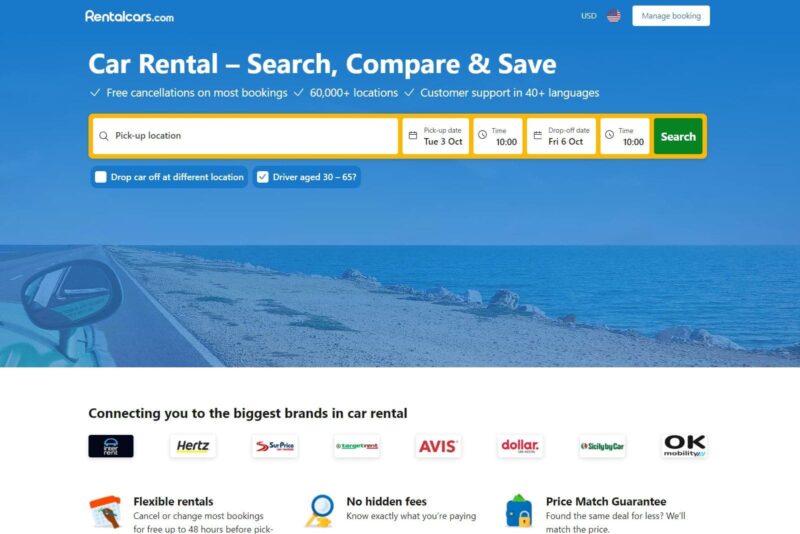Here's a cleaned-up and detailed descriptive caption:

---

This image is a cropped screenshot of the Rentalcars.com website. The header showcases a blue-filtered image of a car driving down a coastal road, giving a serene and scenic backdrop. In the top-left corner, the Rentalcars.com logo is prominently displayed. Towards the right, the currency is set to USD, indicated by both text and a circular icon of the United States flag. Adjacent to it, a white box labeled "Manage Booking" is visible.

Large white typography dominates the center, stating "Car Rental. Search, compare, and save." Below this main heading, a series of checkmarked claims highlight key features: "Free cancellations on most bookings," "60,000+ locations," and "Customer support in 40+ languages."

Further down, search fields for pickup location, pickup date, time, drop-off date, time, and a search button are arranged in a user-friendly format. The lower section of the webpage, set against a white background, declares, "Connecting you to the biggest brands in car rental," with recognizable logos of Hertz, Avis, and Dollar. Below these logos, three boxes enumerate additional benefits: "Flexible rentals," "No hidden fees," and "Price match guarantee."

---

This detailed caption encapsulates all the visual and textual elements present on the screenshot of the Rentalcars.com website.